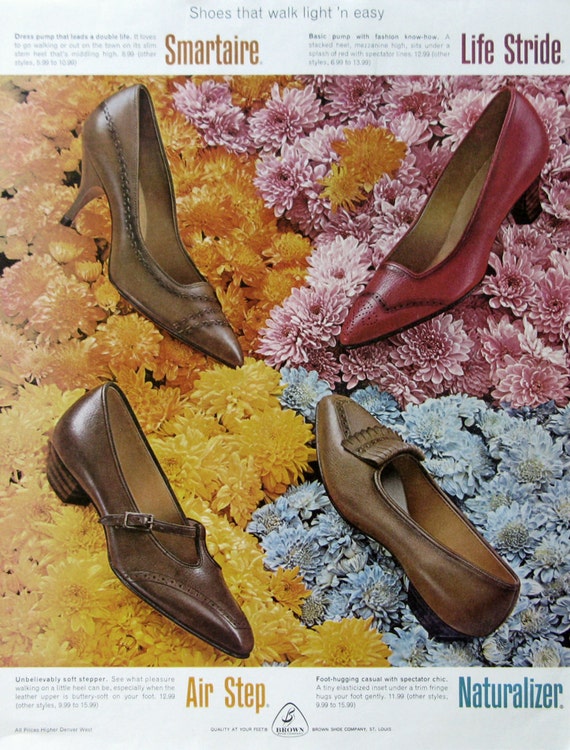This is a portrait-mode advertisement for women's shoes, featuring a total of four distinct leather shoes from different brands. At the top of the ad, on a gray background, it reads "Shoes that walk light and easy." Each shoe is showcased individually with its own floral bedding background.

In the top left corner, the brand "Smart Air" is represented by a lady's high heel shoe placed against a background of peach and orange carnations. Moving to the top right corner, the "Life Stride" brand is marked by a red shoe with a lower heel, set against dark pink carnations.

The bottom left corner features the "Air Step" brand, displaying a brown leather shoe with a single strap and very flat heel, contrasted against its floral bedding. Lastly, the bottom right corner is dedicated to the "Naturalizer" brand, showing a very flat brown shoe adorned with a decorative ribbon at the front.

At the bottom of the advertisement, it states "Quality at your feet" along with the logo for the Brown Shoe Company, based in St. Louis. This nostalgic print ad, likely from the 70s or 80s, combines elegance and practicality, catering to a sense of both style and comfort.